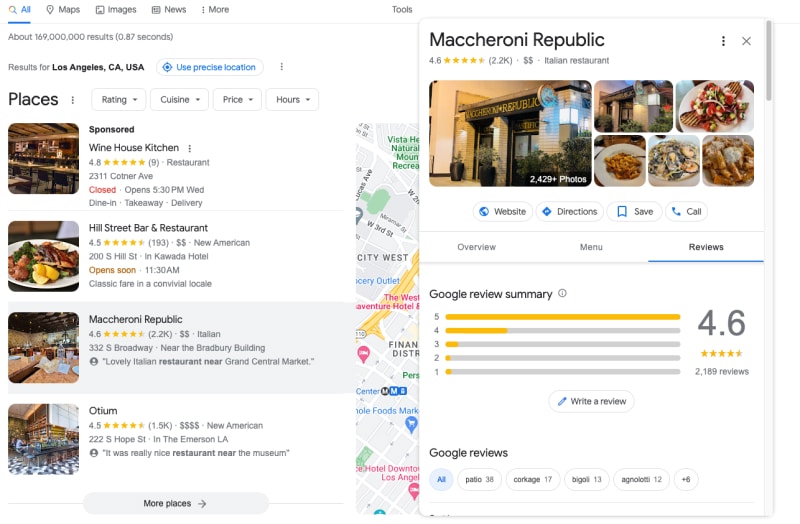A screenshot of a Google search result for restaurants in Los Angeles, California. The image depicts a search page with the "All" button selected and a total of approximately 169 million results displayed in 0.87 seconds. The results include a list of restaurants such as Winehouse Kitchen, Hill Street Bar and Restaurant, Macaron Republic, and Citium.

On the right side of the screenshot, a pop-up window highlights Macaron Republic. The pop-up includes details such as the restaurant's rating of 4.16 stars based on 2.2k reviews, along with images of the restaurant's exterior and various dishes. It's identified as an Italian restaurant. The pop-up also features quick-action buttons for Website, Directions, Save, and Call, and provides a summary of reviews with a 4.6-star rating. The review section includes options for writing a review and searching through Google reviews.

The map is slightly obscured by the pop-up box, indicating the restaurant's location within Los Angeles. Despite some text appearing blurry, additional details about the restaurant are present but not fully legible.